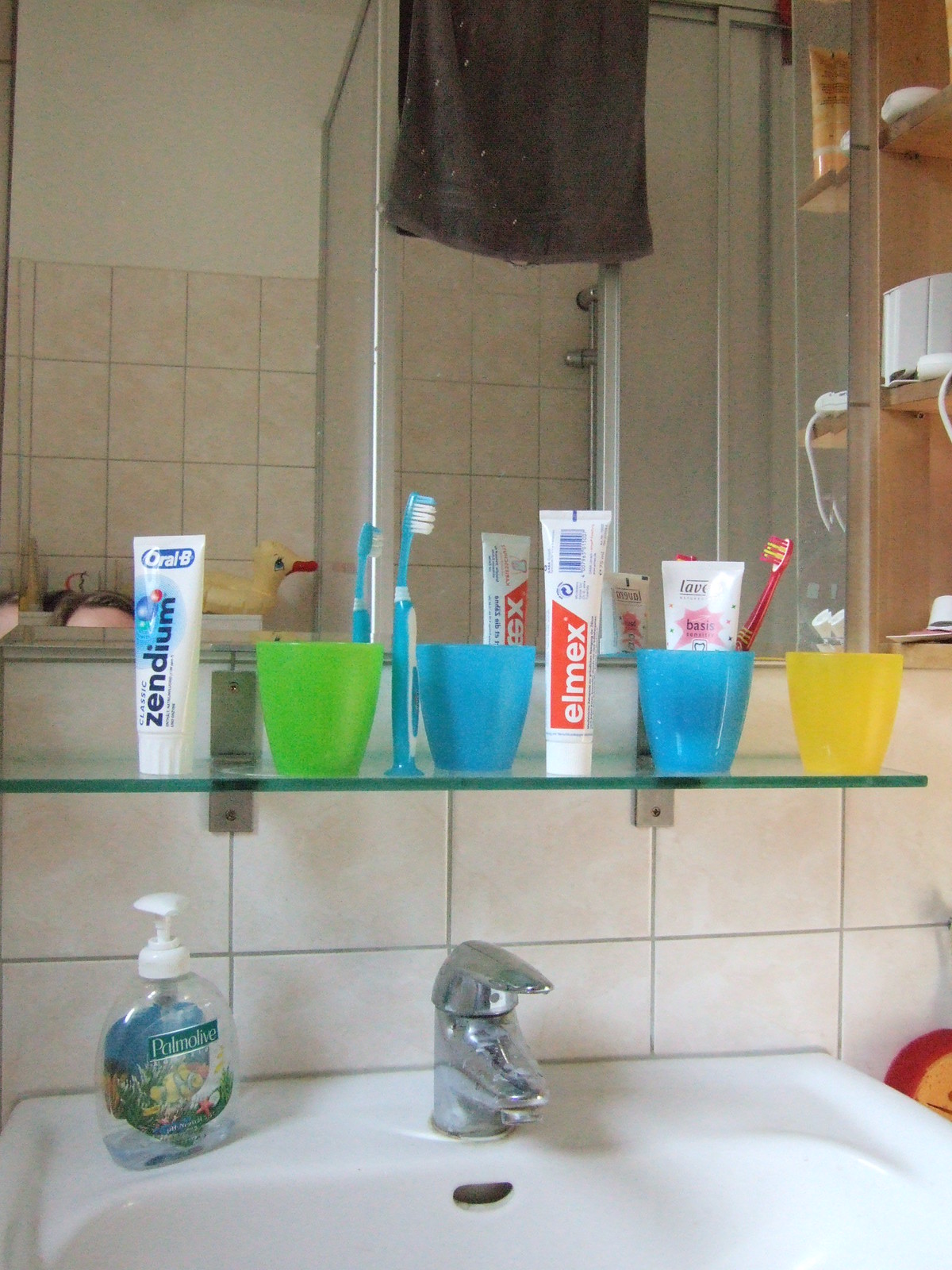The photograph captures a detailed view of a bathroom sink area. Half of the sink is visible, with its white porcelain surface, slightly off-white tiles around it, and a mixer tap featuring a lever-style handle. Adjacent to the tap is a nearly empty bottle of Palmolive clear hand soap with a fish-themed design on its label. Above the sink, a glass shelf houses personal hygiene items: three toothpaste tubes (Oral-B Zendium, and Elmex with its red and white logo), two toothbrushes (one red and one blue), and four rinsing cups (green, blue, blue, and yellow). A mirror behind the shelf reflects these items and part of the scene, including a shower cubicle at the back with a black towel draped over the top. The reflection also captures the very top of a person’s forehead and hair. Overall, the image showcases a well-used, organized bathroom setup.